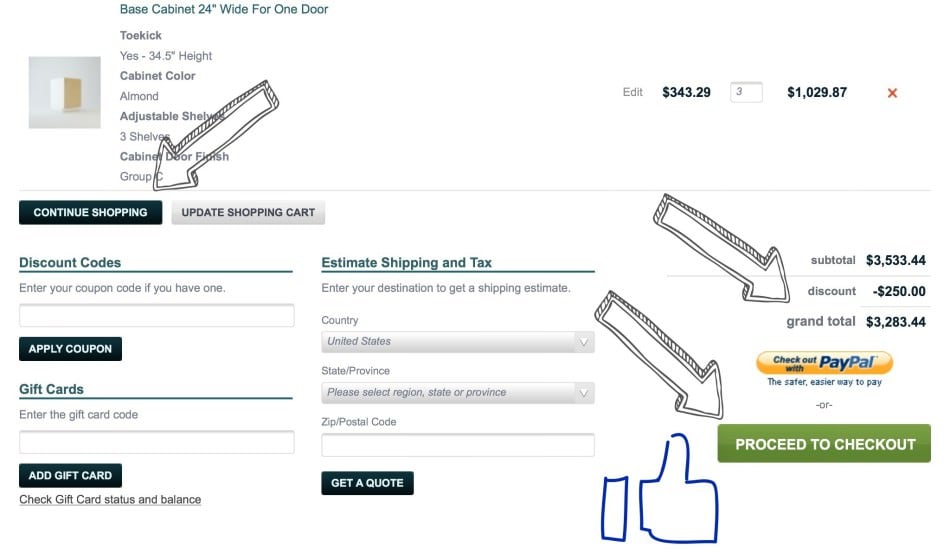In the second image, we see a detailed screenshot of an online shopping cart summary. The focal point is a base cabinet, specifically 24 inches wide with one door, painted blue. Notably, the cabinet is priced at $343.29 each, and the customer has ordered three units, totaling $1,029. 

The interface highlights several key actions with outlined arrows. One arrow points towards the "Continue Shopping" button, another to the "Grand Total" section, and a third directs attention to the "Proceed to Checkout" button. There is also a prominent Facebook-like symbol accompanying the product details, adding emphasis. 

Additionally, the image features a detailed breakdown of costs and options. The subtotal is listed as $3,533.44, with an applied discount of $250. The customer has multiple checkout options, including a standard checkout and a PayPal option. The interface elements are displayed on a white background with blue clickable boxes, contributing to a user-friendly navigation experience.